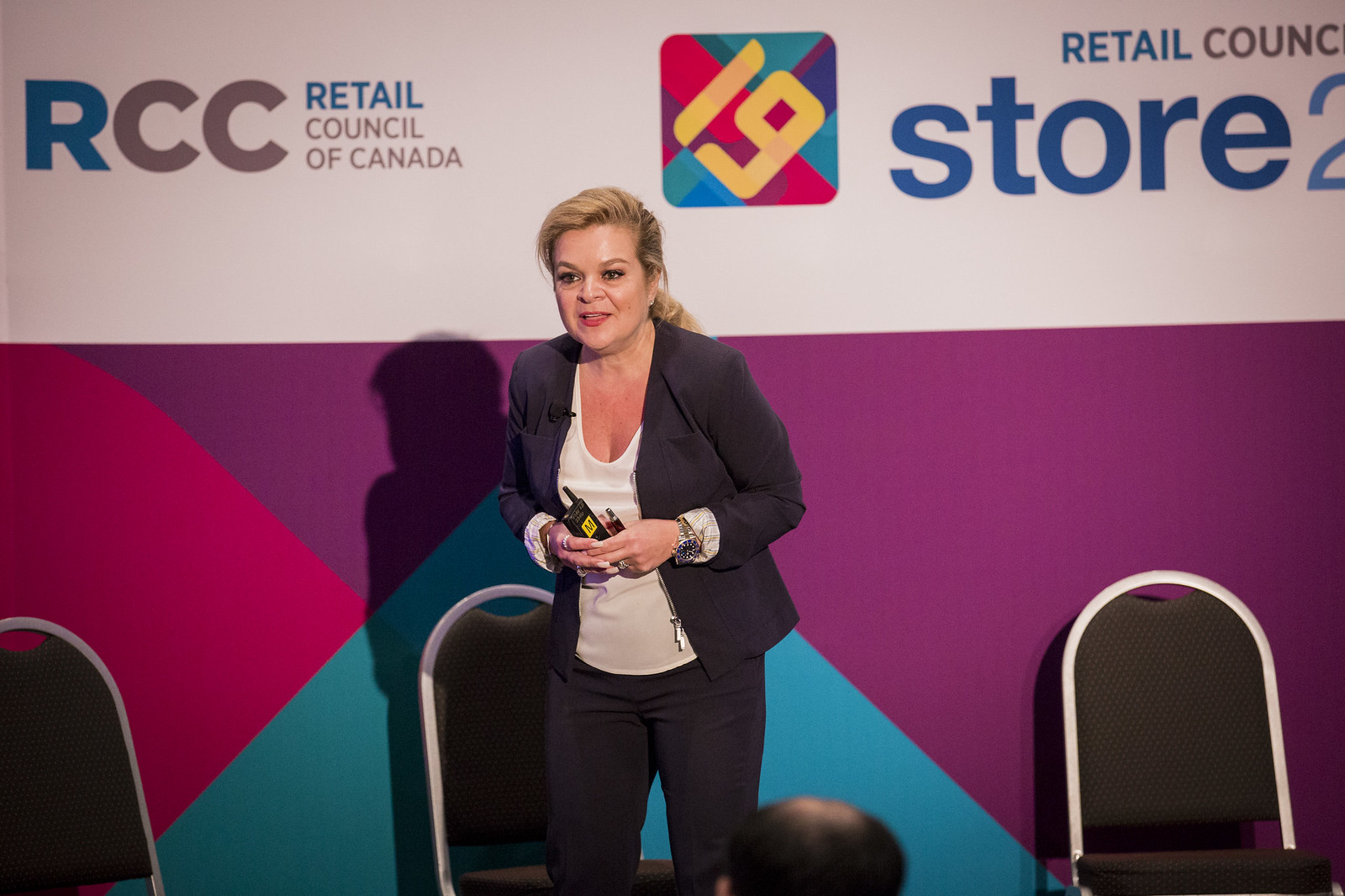In this color photograph with a landscape orientation, a woman stands prominently in front of an audience, partly visible in the foreground. She is positioned on a stage or similar platform, leaning slightly forward, as if speaking to those gathered. The woman, with her long blonde hair pulled back into a ponytail, is dressed in a white blouse paired with a black suit jacket that is open and unbuttoned, and black pants. She holds a walkie-talkie in one hand and a pen in the other. Behind her are three black office chairs with silver metal frames. The backdrop features a banner with the logo "RCC, Retail Council of Canada" in the top left corner, along with the number 19 displayed prominently. The background also showcases geometric designs and additional text elements relating to the Retail Council. The image captures a moment of realistic representation, emphasizing the professional setting and the woman's engagement with her audience.